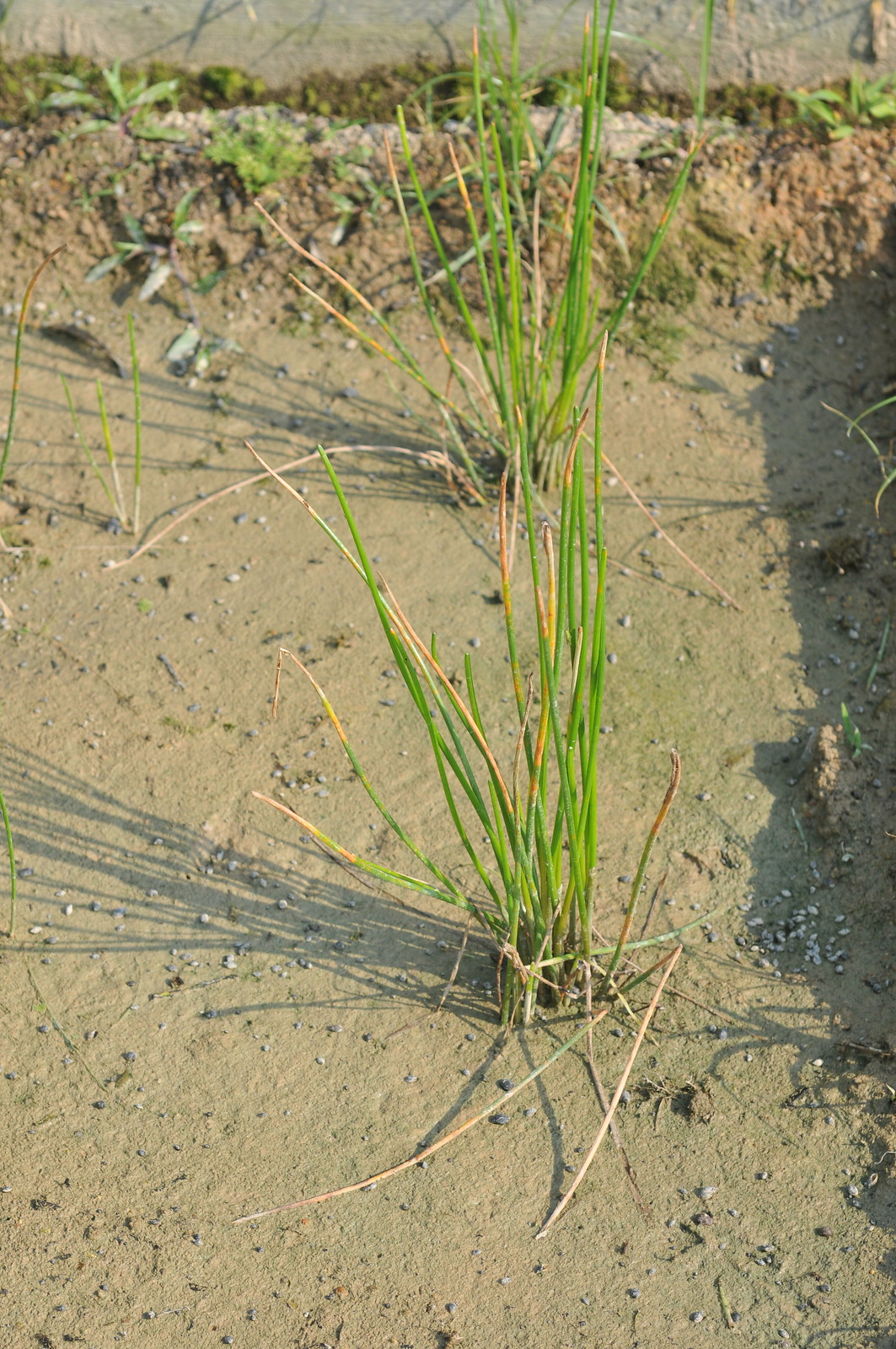The image depicts a beach or similar sandy area, where a notable clump of tall, thin green plants, resembling chives, stands out in the center. This bundle, approximately two feet tall and five inches in diameter, consists of about 30 narrow, string-like strands, each roughly half a centimeter thick. The plants are anchored in a muddy, camel-colored sand substrate mixed with small, grayish-white pebbles and stones scattered around. Behind this central clump, a second similar plant bundle emerges from the muddy ground. Further in the background, there is an earthen mound or border, possibly separating one patch of growth from another. This area is dotted with additional greenery, some weeds, and a bit of rubbish, contributing to a slightly untidy but natural setting. The overall color palette of the scene includes shades of brown and tan, with the shadows indicating that it is a sunny day.